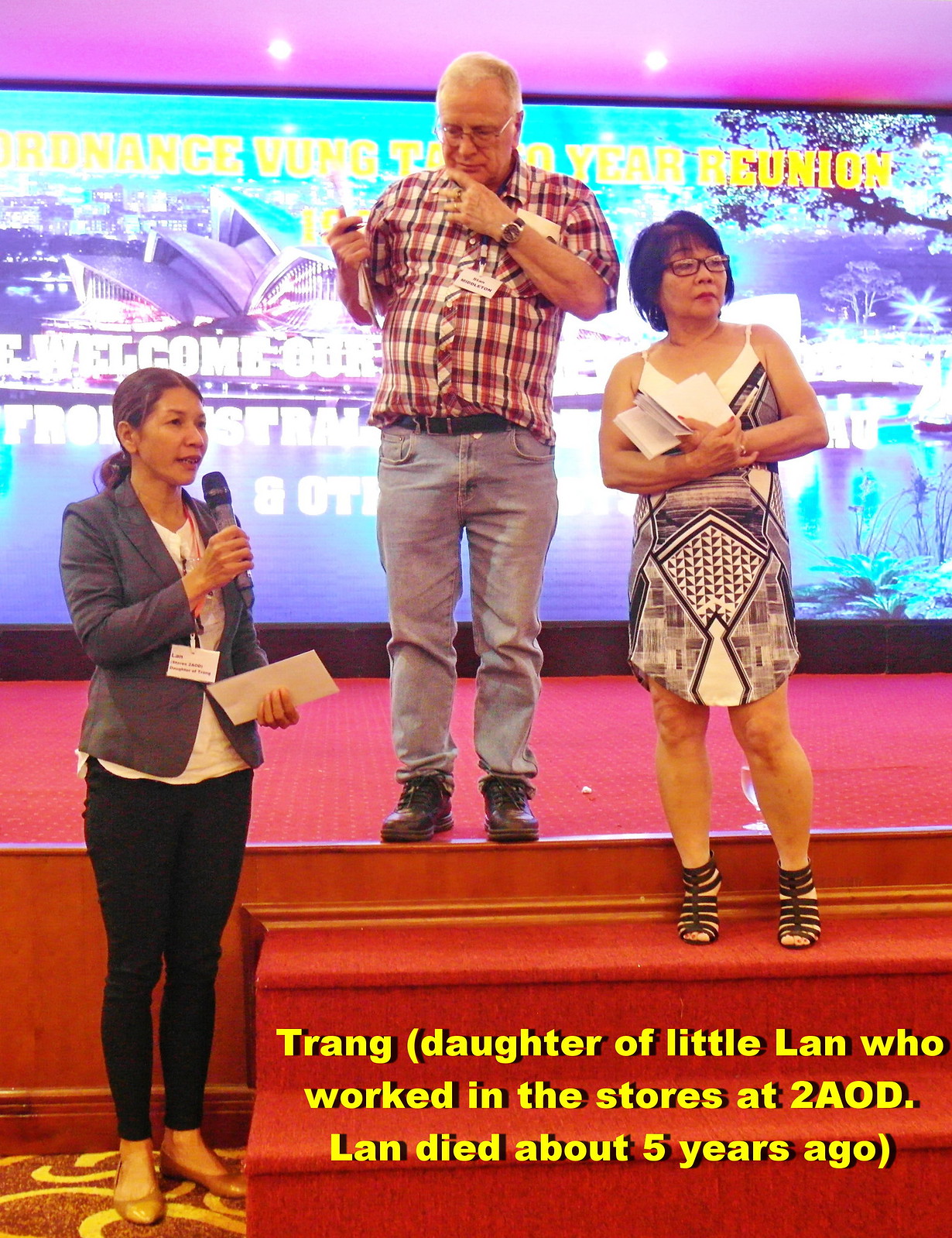The image captures a moment in a room with a stage during what appears to be a memorial or award ceremony, or possibly a reunion in a conference center. At the center of the stage stands a man clad in a plaid shirt, jeans, and a belt, wearing a name tag. To his right, a woman with an Asian appearance is positioned on the red-carpeted stairs leading to the stage. She is dressed in a patterned dress with stripes and sandals wrapping around her ankle. In front of the stage, a woman draped in black leggings, a charcoal gray jacket, and a white shirt is speaking into a microphone. The electronic backdrop prominently features an image of the Sydney Opera House with text in teal, white, and purple hues. A caption in the lower left corner of the photograph reads, "Trang, daughter of Little Lan who worked in the stores at 2AOD. Lan died about five years ago." The combination of their positions, the vivid colors, and the meaningful text suggests a ceremonious gathering marked by remembrance and honor.